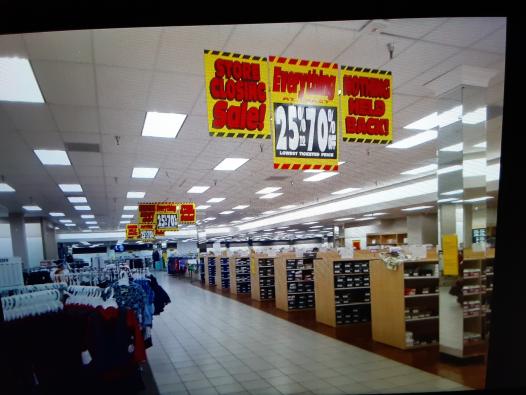The image depicts the interior of a department store that is having a closing sale. At the top of the image, there are three prominent yellow signs with red text announcing the "Store Closing Sale". The central sign emphasizes "Everything Must Go" with a bold declaration, and beneath it, white text indicates discounts ranging from 25% to 70% off. The ceiling is white with a series of white lights receding into the background, creating a sense of depth through perspective.

On the ground, the store features white tile flooring. In the foreground, shelves and display cabinets are arranged, suggesting a shoe department due to the visibly stacked shoe boxes. Towards the left, there are hanging garments, including shirts on white metal hangers, with colors like red and blue prominently displayed. In the background, more clothes and lights are visible, indicating the extensive merchandise available throughout the store.